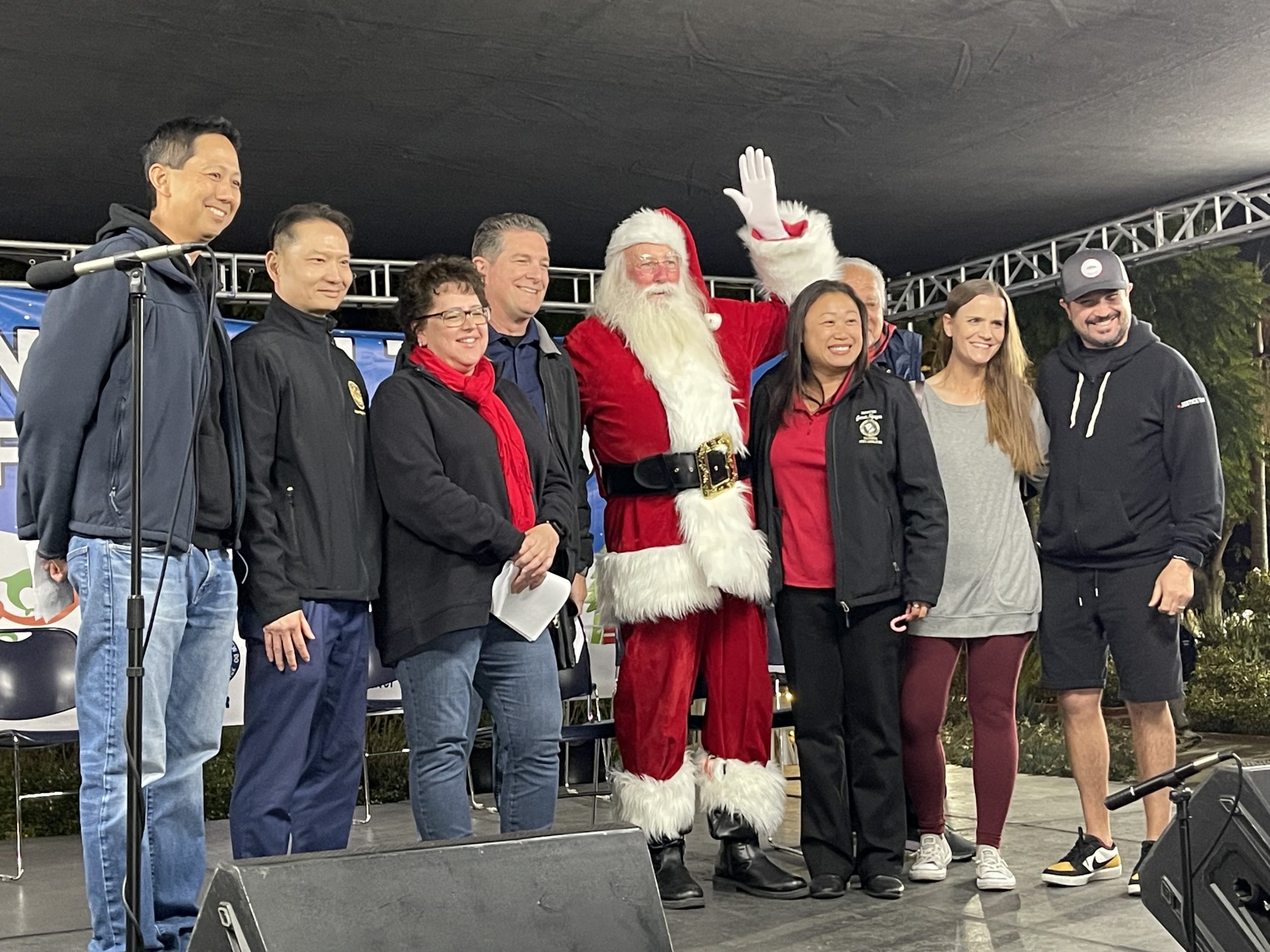The photograph captures a vibrant scene of a group of people standing on an outdoor stage with a black roof supported by metal posts. At the center of the stage stands Santa Claus, dressed in his iconic red suit with white fur trim, a black belt, red hat, and white gloves. He is waving his left hand, and his big white beard and black boots complete the festive look. Surrounding Santa are eight individuals, four on his left and four on his right, all smiling and dressed casually in a mix of jeans, slacks, or leggings paired with sweatshirts, hoodies, or jackets. The person furthest left can be seen wearing a hoodie, baseball hat, and shorts. The stage is equipped with various microphones and loudspeakers pointing towards the crowd, and metal chairs are arranged behind the group beneath a visible banner. This joyful assembly on the makeshift stage captures a celebratory moment with Santa Claus at the heart of the gathering.